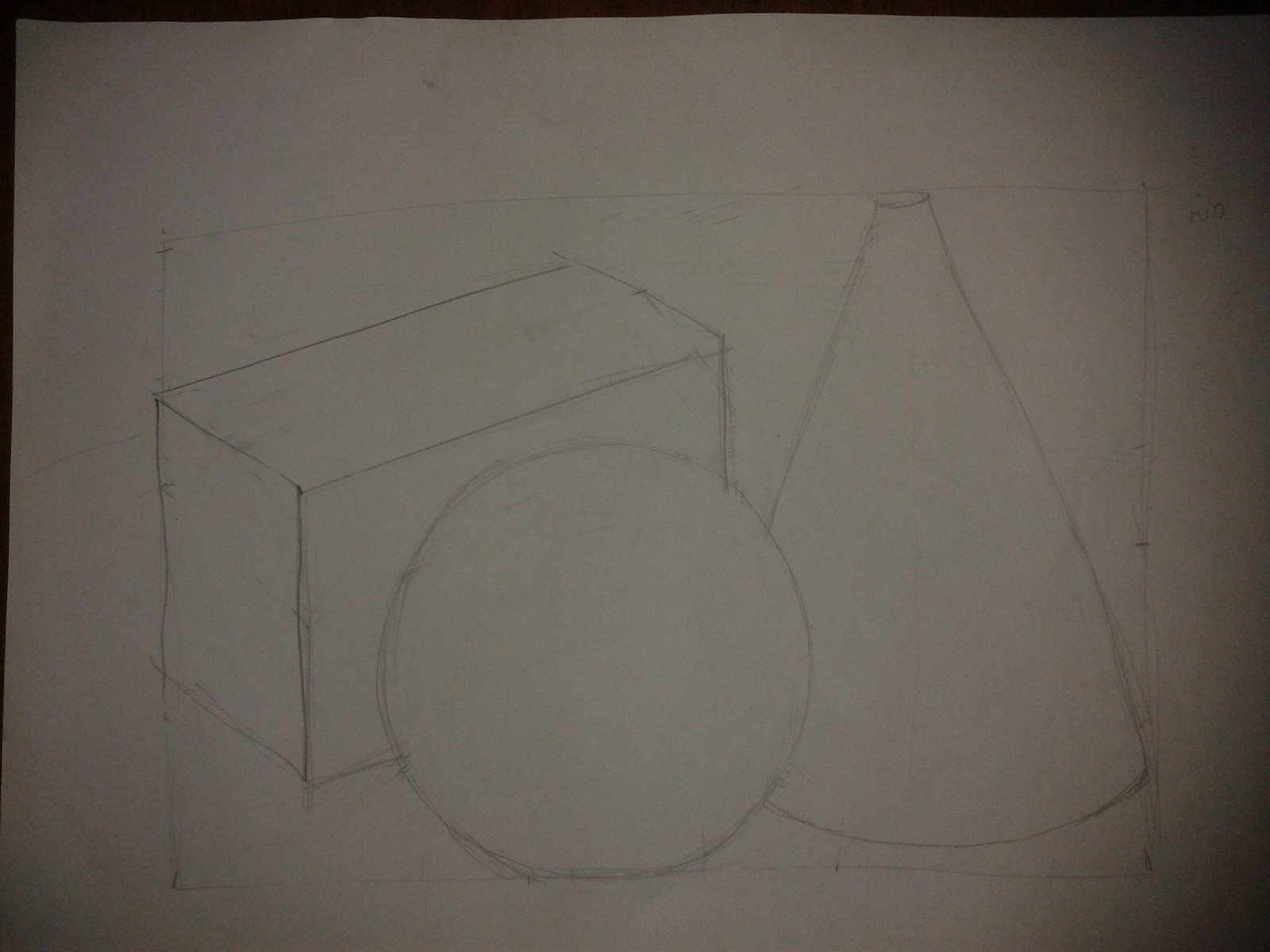This image features a detailed pencil sketch of three geometric shapes arranged within a square outline on white paper. On the left, there is a three-dimensional box angled diagonally, revealing three of its sides. In the center, there is a front-facing circle, and on the right, a front-facing cone. The sketches are done with fine, delicate lines, and the image appears to be closely zoomed in. The top portion of the image showcases an abstract black background, creating a striking contrast that highlights the intricacies of the sketched shapes.